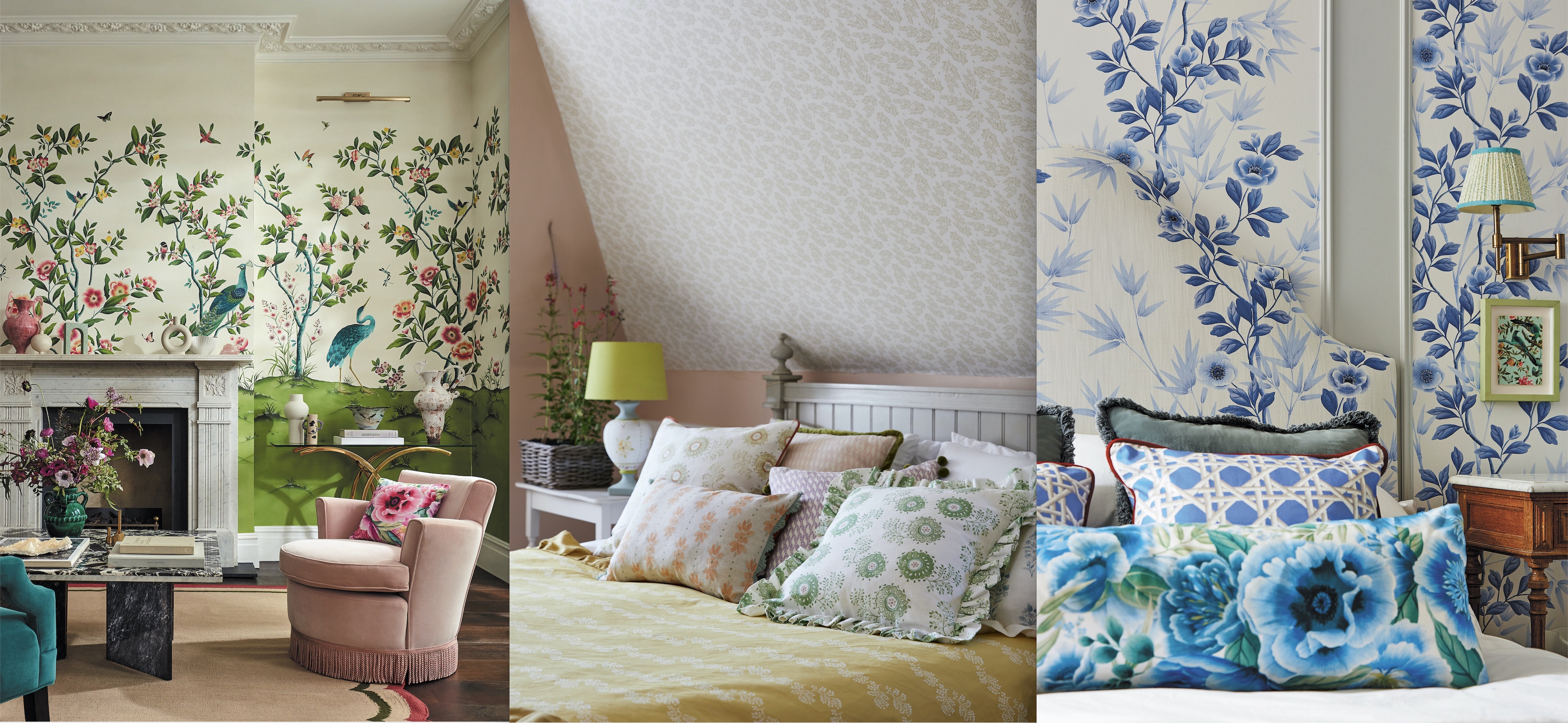This image features three adjacent interior designs, each highlighting distinct room styles. The left section depicts a charming living area with a beige wallpaper adorned with pink and blue flowers intertwined with green vines. A central white-framed fireplace anchors the room, flanked by a teal chair on the left and a muted pink chair with a pink floral pillow on the right. Between these chairs lies a coffee table adorned with pink flowers in a vase. The middle section reveals a quaint bedroom resembling an attic space with slanted walls. This bedroom features a white and pink color scheme with a unique feather-textured white wallpaper on the vaulted sections. The bed, framed in light wood, is dressed with a yellow comforter and assorted colorful floral pillows. A white bedside table supports a lamp with a celery green shade, beside which stands a plant in a square pot. The right section showcases another bedroom with blue floral wallpaper set against a white background. The bed has a white comforter and is piled high with an array of blue-patterned pillows. The headboard and walls are cohesively decorated with the same blue vine and flower motif, complemented by a white lamp with blue trim that extends from the wall.